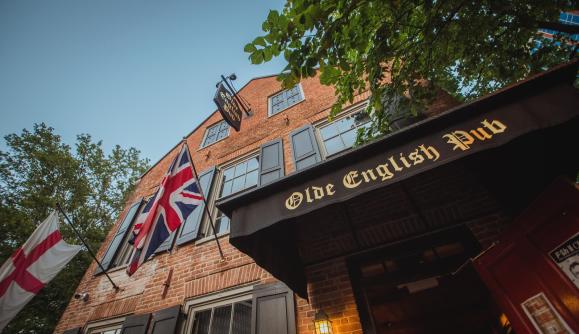The photograph is taken outdoors during the daytime, capturing a three-story, well-maintained, old brick building, probably located in England. The building is rectangular in shape and constructed of reddish-brown bricks. The view is angled upwards, beginning with a brown door at the lower right-hand corner, just beneath a dark brown wooden awning or overhang which bears the gold-lettered inscription "Olde English Pub." Above this overhang, a green-leaved tree extends into the upper right corner. Blue sky is visible in the upper left. Central to the image, protruding from a pipe near the top of the building, a wooden sign also reads "Olde English Pub." The facade features multiple windows: two at the top, three in the middle, and at least two at the bottom, all framed with modern shutters. Flying above the building are two flags; the one on the left with a white background and a red cross, possibly the flag of England, and the other, slightly higher and more central, is the Union Jack. Adding a quaint touch, a gaslight fixture is positioned next to the entrance at the bottom left.